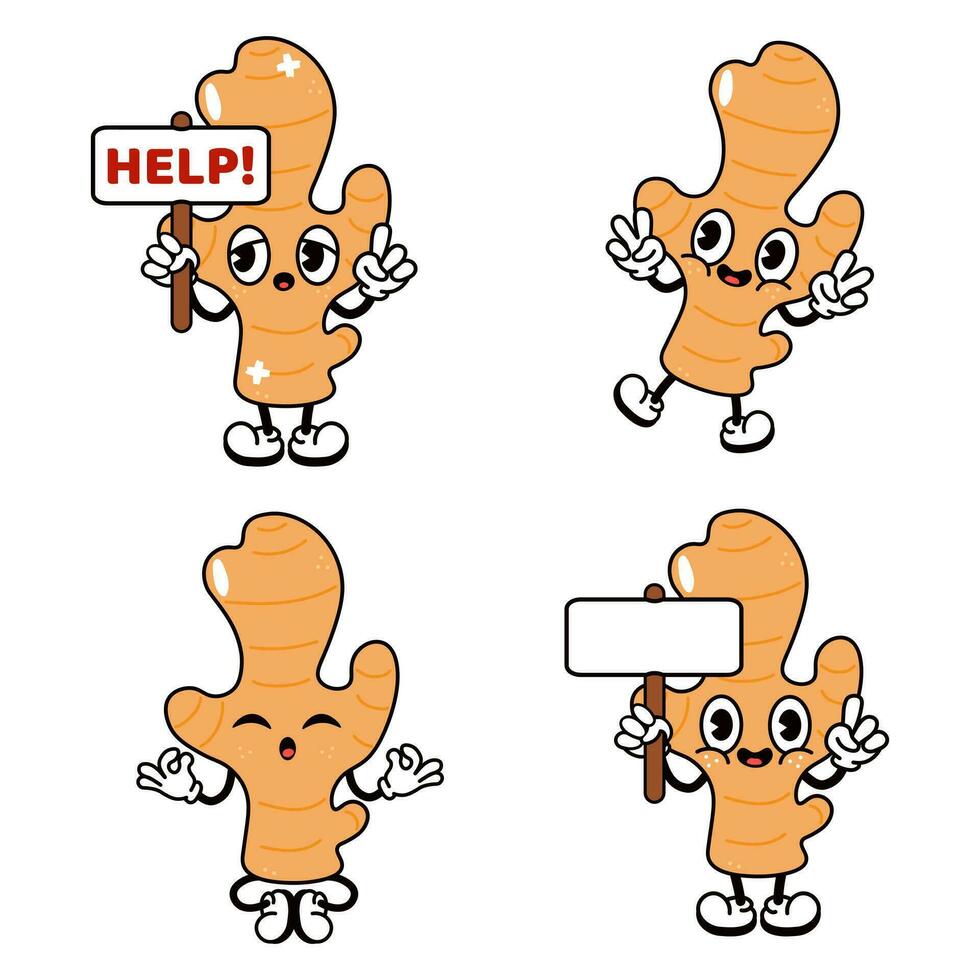This cartoonish illustration features a sequence of four ginger root characters, each in a distinct pose and expressing different emotions. All the ginger roots have a light brown color with darker brown horizontal stripes, giving them a distinctive textured look. They all share similar cartoonish features, including large black-pupil eyes, a small black mouth, white gloved hands, and white shoes attached to thin black legs.

In the top left cell, the ginger root looks distressed with bandages on its head and lower right body. It holds a wooden stick with a white sign bearing the word "HELP" in red text. The eyes convey a sense of desperation, and a pink tongue is visible in its small mouth.

To the right, in the top right cell, the ginger root appears cheerful, smiling broadly while holding up both hands in peace signs.

The bottom left cell features the ginger root in a meditative pose, with eyes closed, legs crossed, and hands positioned with index fingers and thumbs touching.

Finally, the bottom right cell showcases a very happy ginger root, smiling widely with three freckles on each cheek. It holds up both hands and displays a blank white sign similar to the one in the first cell.